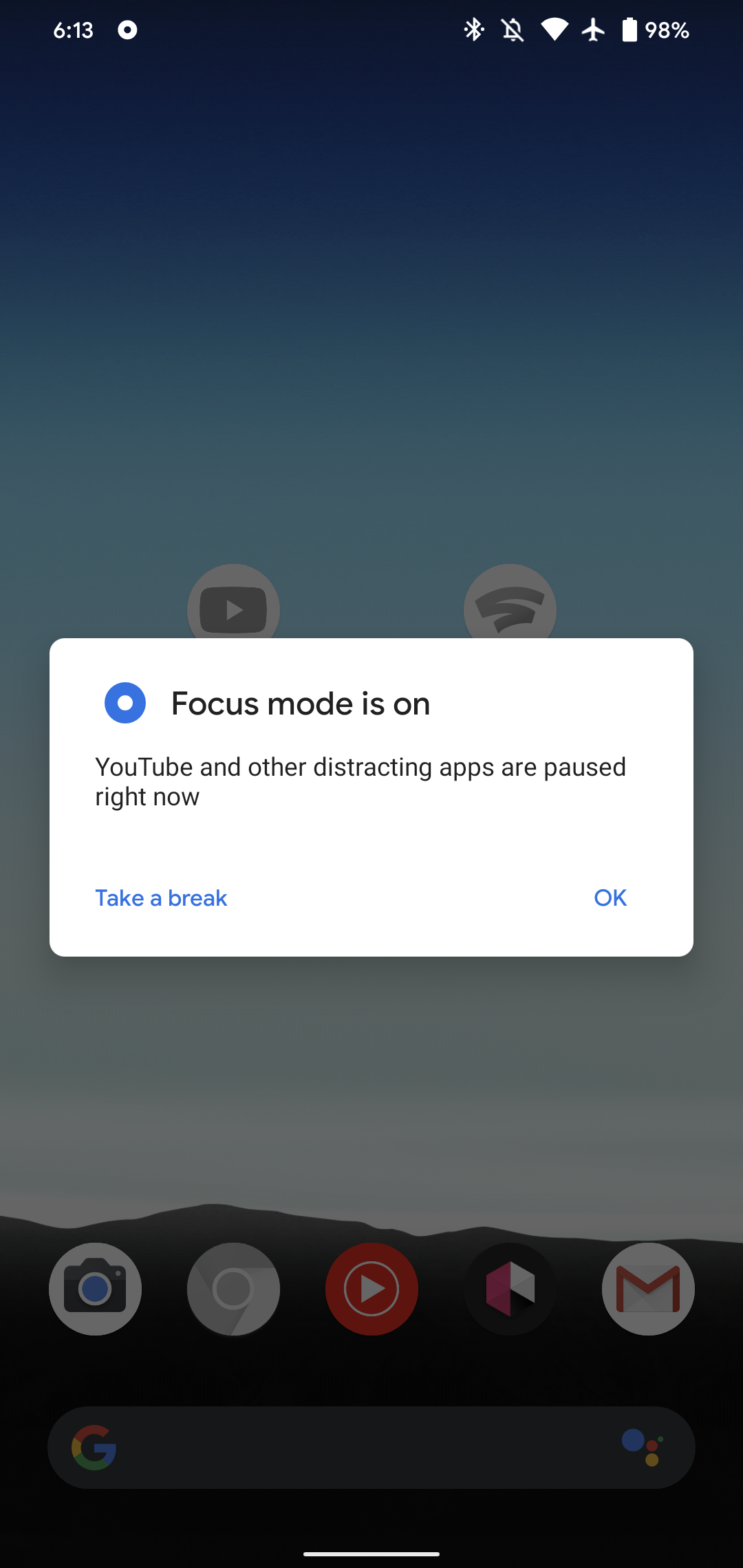A detailed digital depiction of a cell phone screen is shown, though the phone itself is not visible. In the upper left corner, the time is displayed as 6:13. The upper right corner includes several icons indicating that Wi-Fi is enabled, no notifications are present, airplane mode is activated, and the battery is charged at 98%. The background gradient transitions from a dark blue at the top to almost white at the bottom, where a silhouetted hill or mountain arises.

Aligned on the hill are several application icons, likely including those for a phone, Google, YouTube, an unidentifiable app, and Gmail. Below these icons, a Google search bar with an AI icon appears, slightly grayed out. Superimposed on this is a white, horizontally elongated rectangle with a message stating, "Focus mode is on. YouTube and other distracting apps are paused right now." Underneath this message, there are two options: a blue link labeled "Take a break" on the left, and "OK" on the right. The color palette features shades of white, blue, black, red, pink, yellow, green, and gray.